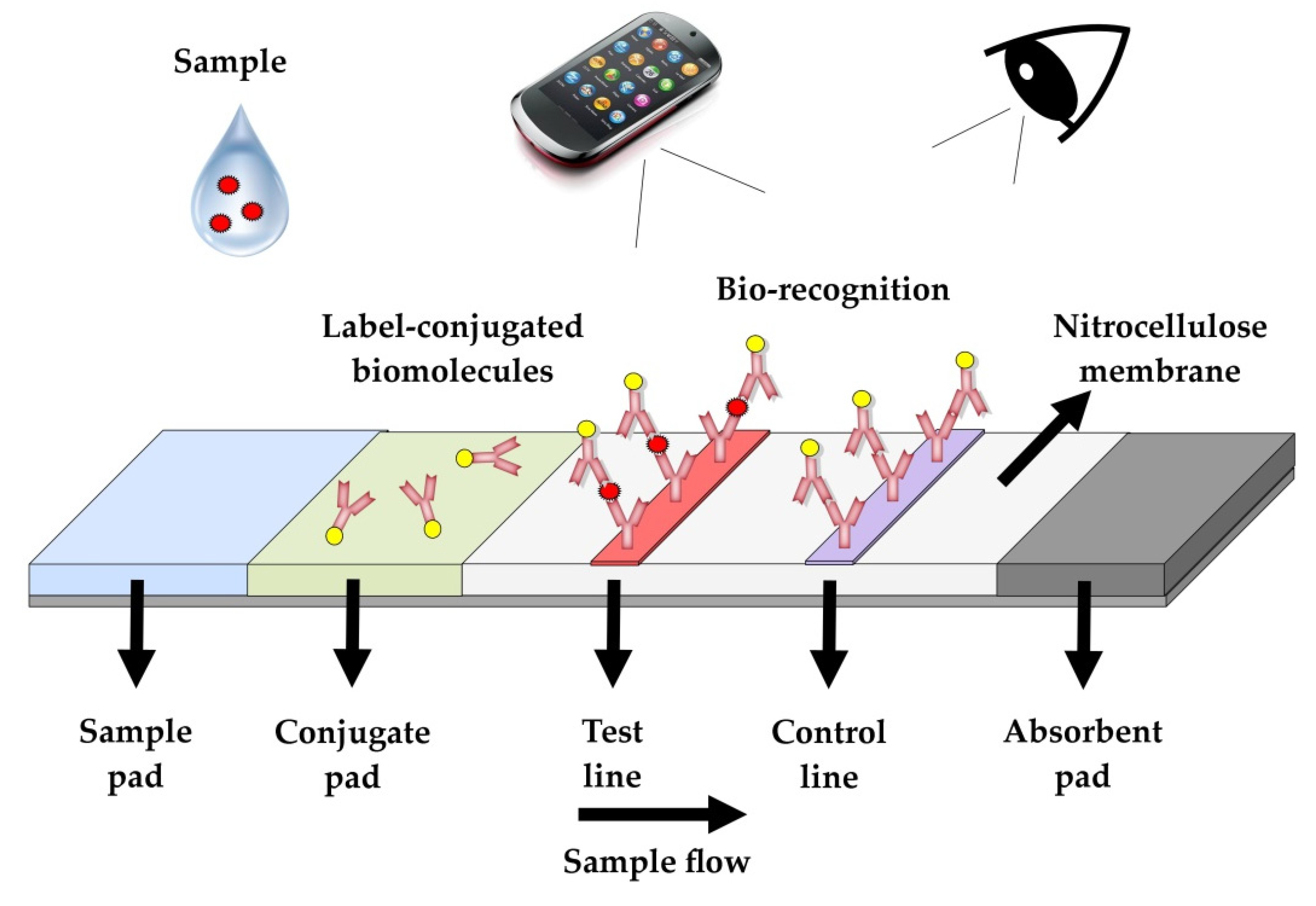This is a highly detailed instructional diagram presented on a white background. The diagram starts at the top with an image of a clear water droplet containing three red circles, labeled "Sample." Adjacent to this is an illustration of a smartphone with two lines extending from it, and then an eye with two lines extending from it. Above these images are the labels "Sample," "Label Conjugated Biomolecules," "Biorecognition," and "Nitrocellulose Membrane."

The main section of the diagram features a horizontal oblong pad divided into five distinct color-coded sections, each with its own label and additional symbolic illustrations. From left to right, the sections are as follows:

1. **Sample Pad**: A blue section marked "Sample Pad," with a black arrow above pointing downwards.
2. **Conjugate Pad**: A green section labeled "Conjugate Pad," adorned with numerous pink stick-like figures topped with yellow dots.
3. **Test Line**: A white section featuring a prominent red line labeled "Test Line," with the same stick-like figures now standing upright.
4. **Control Line**: A light purple section labeled "Control Line," also populated with the upright stick figures.
5. **Absorbent Pad**: A gray section labeled "Absorbent Pad."

Above these sections, there is a line representing the sample flow, guiding through the process starting from the water droplet sample, past the smartphone and eye icons, finally moving through each colored section. Below, extending from one of the white sections is a line labeled "Nitrocellulose Membrane." This thorough and visually detailed diagram illustrates the procedural flow of the sample through various stages, indicating the absorption, reaction, and containment carried out at each pad and line.